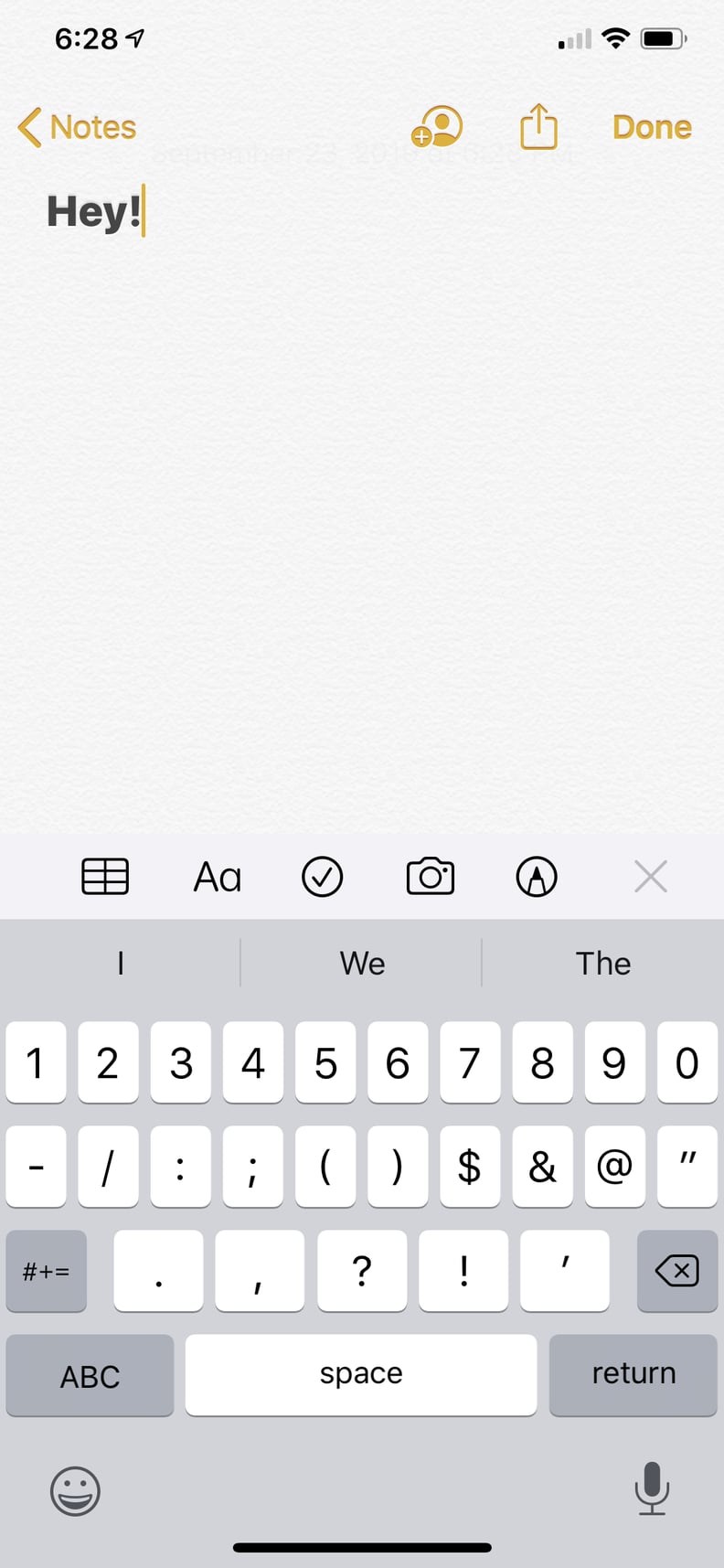In this image, the background is a light purple color. At the top center, the timestamp reads "6:28." Dominating the upper part of the image, a blue arrow points upward and to the right, while a yellow arrow points to the left and is accompanied by several musical notes. Near the center, a small person icon appears inside a yellow circle containing a dot with a plus mark. To the right of this icon, there's a square containing an upward-pointing arrow next to the word "Done."

Overlaying the light purple background, someone has handwritten the word "Hey" with a small yellow mark accentuating it. Beneath this, the background transitions into a darker purple section, featuring a smaller black box with a diagonal line running through its middle, segmenting it into three sections on each side. Adjacent to this box are icons of a large and small "A," a circle with a checkmark, a camera, a circle with a pen tip, and an "X." 

The image also includes a keyboard layout. The keyboard keys are white with black characters and symbols. At the top, the words "I," "We," and "@" are displayed. On the lower-left side of the keyboard, there's a purple button labeled "#+=" and another labeled "ABC." The space bar is situated in the lower middle. On the right side, there is a purple return button, and just above it, a purple button with a black square and an "X" inside it.

At the very bottom in light purple, a small smiley face and a microphone icon are visible, accompanied by a black horizontal line. This line appears to separate the image into distinct sections.